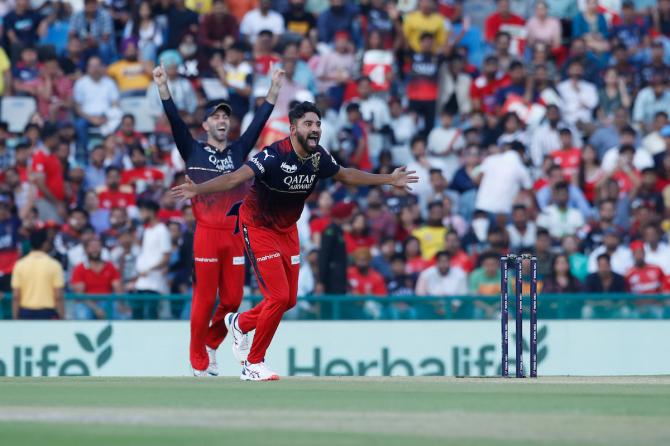The image is a full-color photograph taken outdoors, likely at a cricket stadium, during the daytime using natural light. The scene is at ground level, focusing on a cricket field. At the center of the field, two South Asian men, possibly South Indian, are celebrating. These players are wearing black jerseys with "Qatar Airways" written on them, long red pants with the text "M-A-H-I-N-D-S" or similar, and white sneakers. One man has both of his hands raised, while the other has his hands stretched out. 

Three upright cricket bats can be seen in the bottom right of the image, identifying the sport. The field around them is green and white. 

In the background, a partially blurred crowd of predominantly South Asian spectators is visible, many dressed in white and red shirts. Behind the crowd, a banner with "Herbalife" or "Herbal Life" can be spotted, along with another sign that reads "Urban Life."